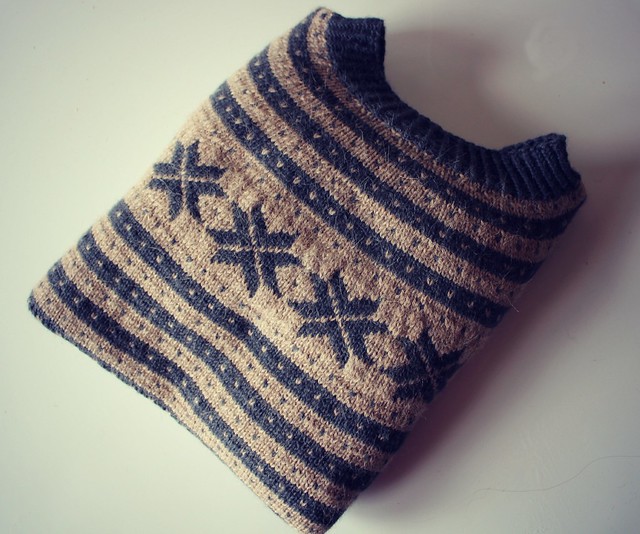This image features a neatly folded, knitted sweater displayed on a light gray or white surface, with its shadow subtly cast onto the background. The vantage point looks directly down at the sweater, giving no indication of the edges of the surface it rests on. The sweater, folded into a compact square and tilted slightly to the right, prominently displays its front. It features a blue crew neck collar, and primarily consists of alternating stripes in a dusty blue and tan palette. The central, broader stripe across the chest is a pale tan, adorned with blue, stylized star or snowflake patterns, contributing to a festive or possibly Christmas-themed aesthetic. This particular layout is reminiscent of product display images you might find on Pinterest or Etsy, emphasizing the sweater's design and tidy presentation.